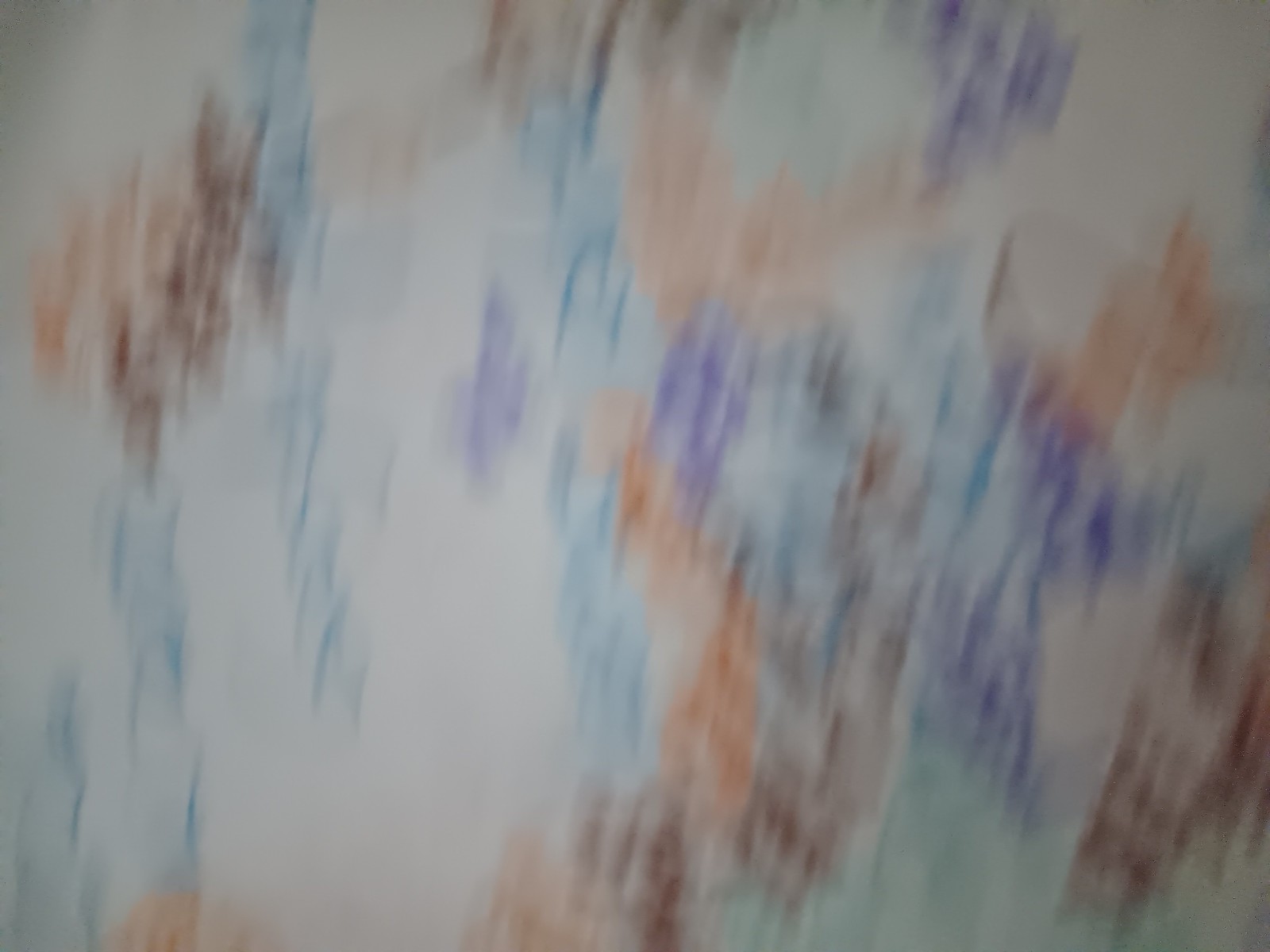This is a very blurred image of what seems to be a drawing on a flat, white surface. The drawing features a chaotic array of randomly distributed multicolored sections. The colors, including dark brown, orange, light blue, royal purple, white, red, yellow, cyan, and possibly light green, appear in a pattern resembling random blobs or crosshatches, suggesting the medium might be crayon or something similar. The blurred appearance gives the impression of a photo taken either in motion or without proper lighting, making the colors look faded. The image evokes the thought of a child’s drawing, with no discernible text present.